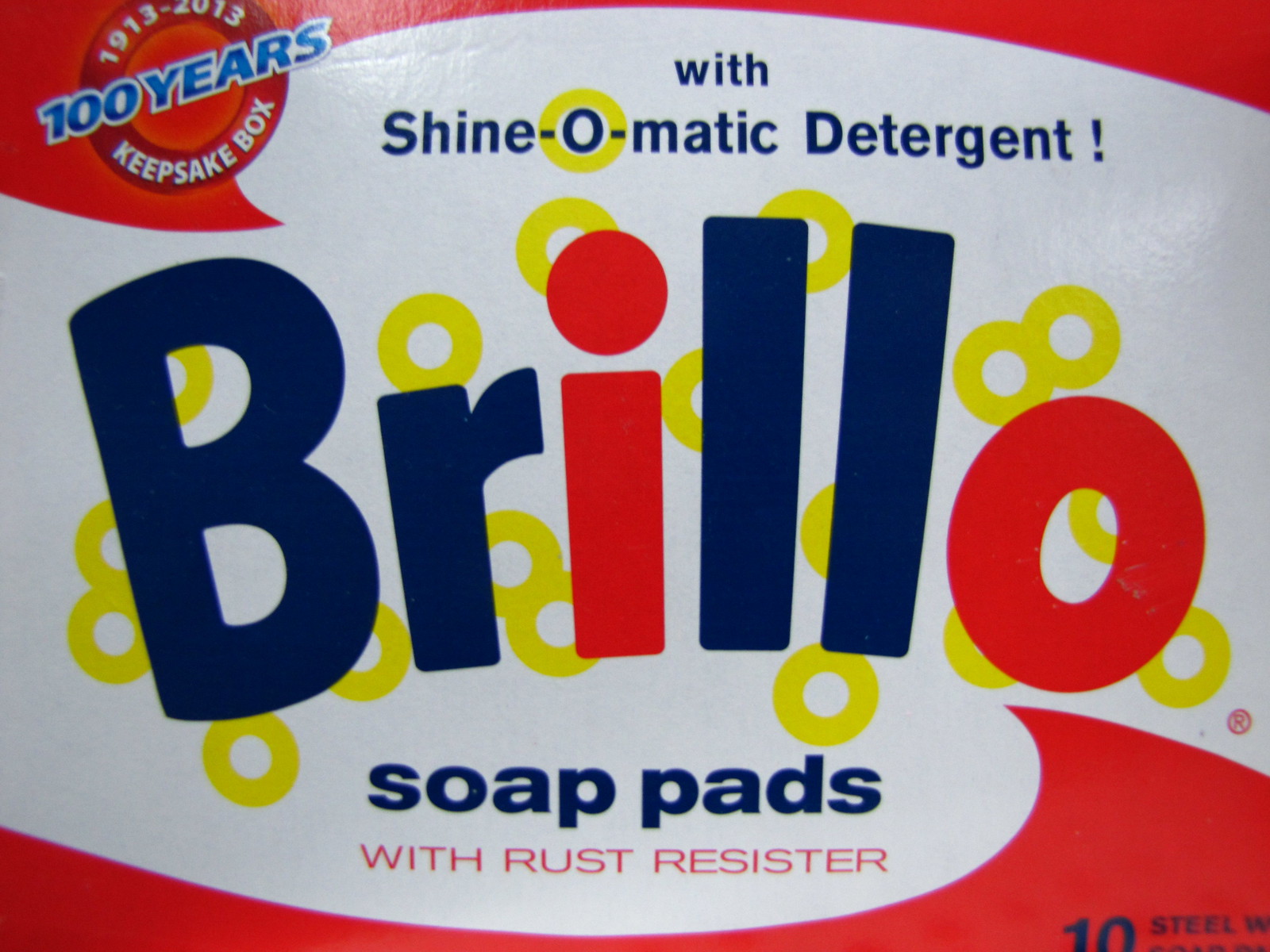This image is a close-up of a commemorative box of Brillo soap pads celebrating their 100th anniversary from 1913 to 2013. Dominated by vibrant colors, the design features a striking combination of red, blue, yellow, and white. At the top left corner, a circular badge marks the anniversary with the years "1913-2013" in blue and the words "keepsake box" at the bottom of the circle. Adjacent to this, in small blue text, reads "with Shinomatic detergent."

The central focus is the prominent Brillo logo. The letters “BR” and “LL” are in bold blue, while the “I” and the final “O” are in bright red. The “O” is uniquely highlighted with yellow circles resembling the number 8, adding a playful yet dynamic element. Beneath the Brillo name, in blue letters, the box states "soap pads," followed by a smaller red inscription that reads "with rust resistor." A red wave design elegantly frames the top and bottom of the image, adding a visual balance. The bottom right corner partially shows additional product information, indicating "10 steel wool pads." The overall composition and text placement emphasize the brand's historic milestone while maintaining a cohesive and eye-catching design.